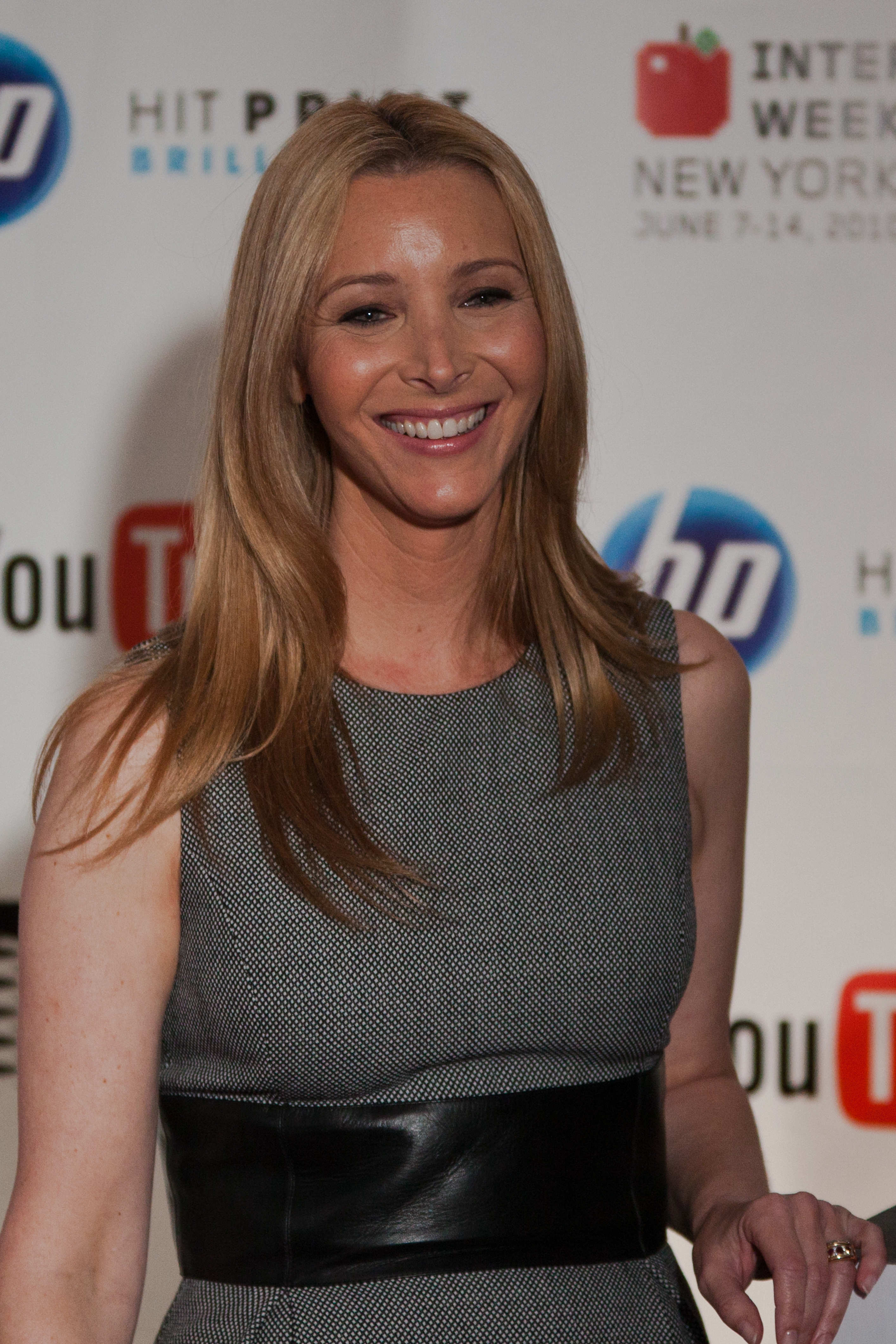This photograph captures Lisa Kudrow standing in front of a white banner adorned with various business logos, including YouTube and HP, with one partially obscured logo. Lisa is dressed in a stylish gray and black tank top-style dress featuring a pattern of very small checks. The dress is cinched at the waist with a prominent leather belt. Her signature thin blonde hair falls to her shoulders, and she wears a genuine, full smile directed slightly off-camera. Her bare arms and shoulders are visible, and she wears a single gold ring on her left hand, which appears to be resting on an unseen object to the side. The photo, taken from the waist up, showcases Lisa Kudrow at an event, capturing her elegance and joyful demeanor.